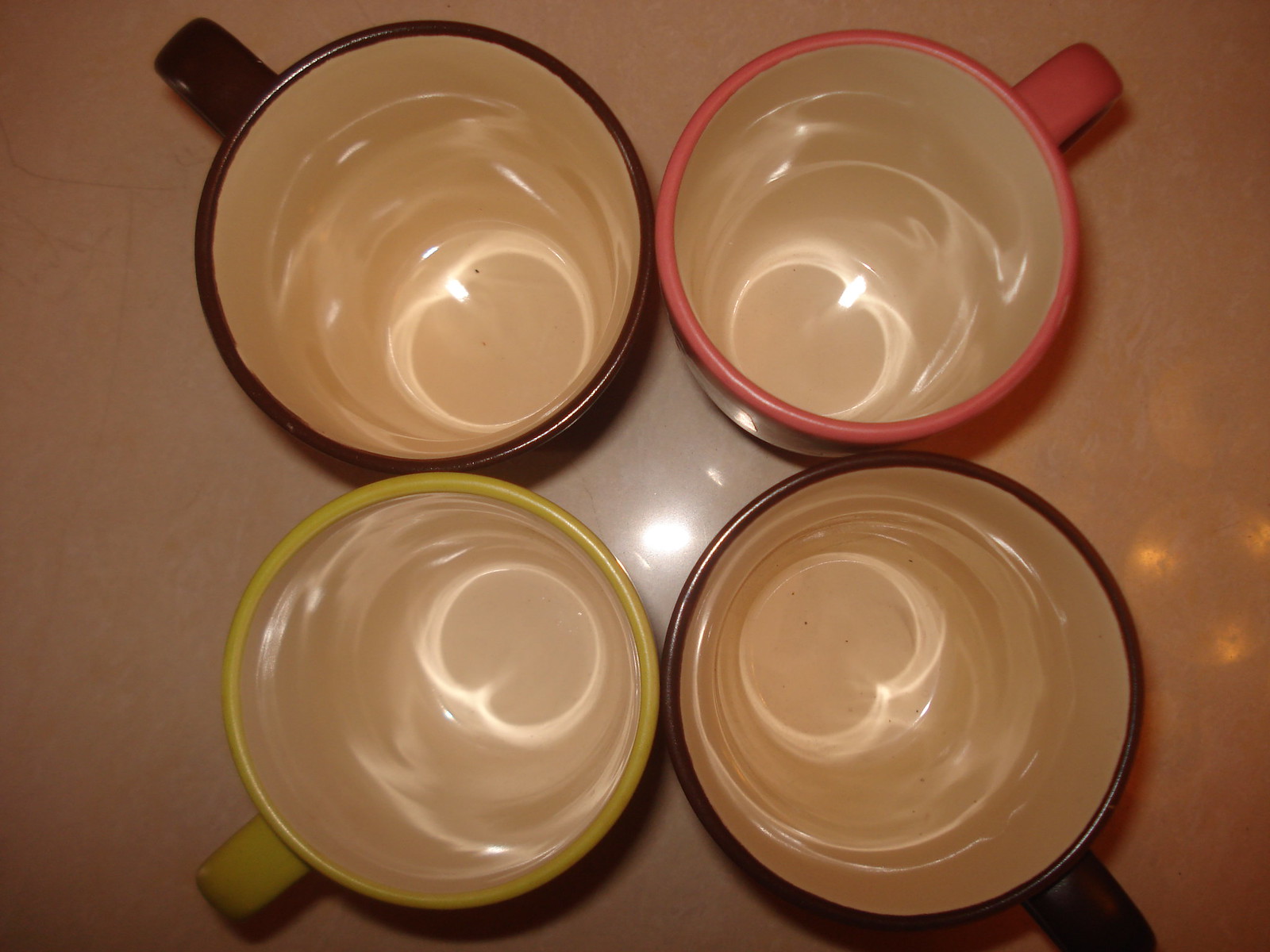This overhead close-up view shows four ceramic coffee mugs arranged in a tight square formation on what appears to be a shiny, pale brown or possibly white surface. The mugs, touching at the rims and creating an X shape with their handles pointing outward, are lit from above, causing bright reflections inside their off-white interiors. The top left mug is a deep brown or black with its handle facing the upper left corner, while the top right mug is a bright orange or possibly pink with the handle pointing to the upper right. Below the brown mug, in the lower left, is a vivid yellow mug with its handle directed downward. Adjacent to the yellow mug, at the bottom right, is another dark-hued mug, either brown or black, matching the diagonal counterpart, with its handle also pointing downward. Each mug appears to be of similar size, around 20 ounces, and the surface reflects the light, adding to the overall shine of the composition.